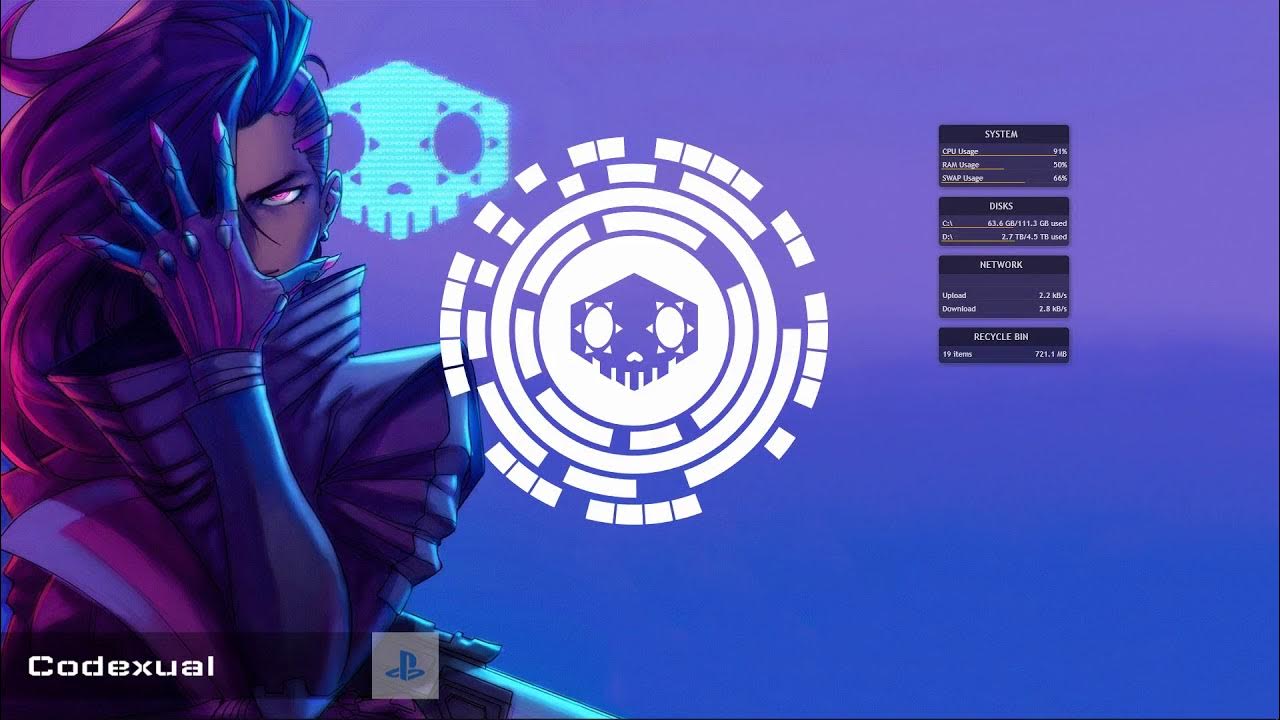The image features a digital illustration with a gradient purple background, which transitions from lighter purple at the top to a darker shade at the bottom. Dominating the left side is an animated female character, dark-skinned with striking blue and purple hair featuring bright pink tips. Her hair, styled with one side shaved, falls flowingly over her face, partially obscuring one pink eye with her hand. She wears an intricate, tight purple outfit adorned with padded, pointy shoulder pieces and a samurai-inspired collar. Her hands are equipped with purple gloves ending in pointy tips resembling claws, similar to Wolverine's but without extending spikes.

In the center of the image, there is a prominent white circular logo with a stylized purple skull in the middle. Surrounding the skull are concentric circles with intermittent breaks, and small white triangles are arranged around the skull's eyes. 

On the right side, there are displayed system statistics under the headings 'System,' 'Discs,' 'Network,' and 'Recycle Bin,' showing details like 91% CPU usage, 50% RAM usage, 66% swap usage, disk usage of 66.6 GB with 2.7 TB out of 4.5 TB used.

In the bottom left corner of the image, the text "Codexual" is displayed alongside a PlayStation logo (P.S.).